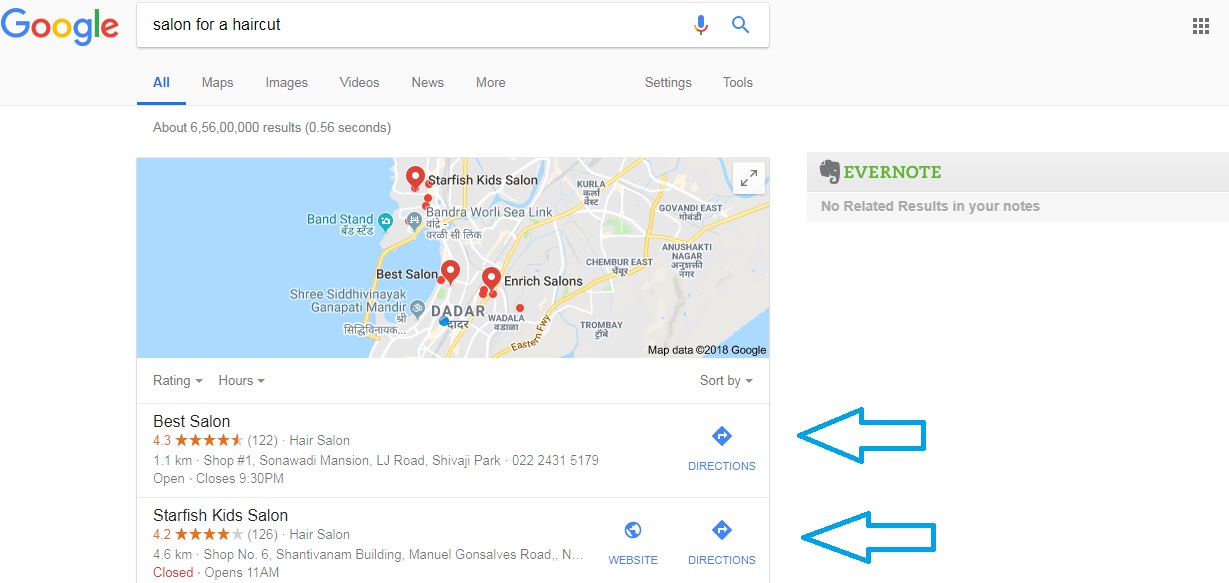Google Search Results Page for "Salon for a Haircut"

At the top left corner of the page, the word "Google" appears in its traditional colors: blue, red, yellow, and green. To the right of the logo is a white search box containing the phrase "salon for a haircut." Adjacent to the search box on its right, there are two icons inside: a microphone and a magnifying glass. This entire section is set against a very pale gray ribbon that runs horizontally across the page.

Directly below this ribbon, still within the pale gray area, are several navigation options: "All," "Maps," "Images," "Videos," "News," and "More." Towards the far right of this ribbon are the "Settings" and "Tools" options.

The main body of the screen displays a predominantly white background. At the top of this section, in small gray text, it states that approximately 6 million results were found in 0.56 seconds. 

Beneath this text, there's a map illustrating the query results. The map features a light gray background with roads highlighted in white and major highways marked in gold, all appropriately labeled. Three locations are pinned with the red location icon. To the left of the landmass depicted on the map, there is an unlabeled body of water.

Following the map, two search results are shown in a vertical list:
1. **Best Salon** - includes a star rating, address, hours of operation, and directions.
2. **Starfish Kids Salon** - includes a star rating, address, hours of operation, directions, and a link to its website.